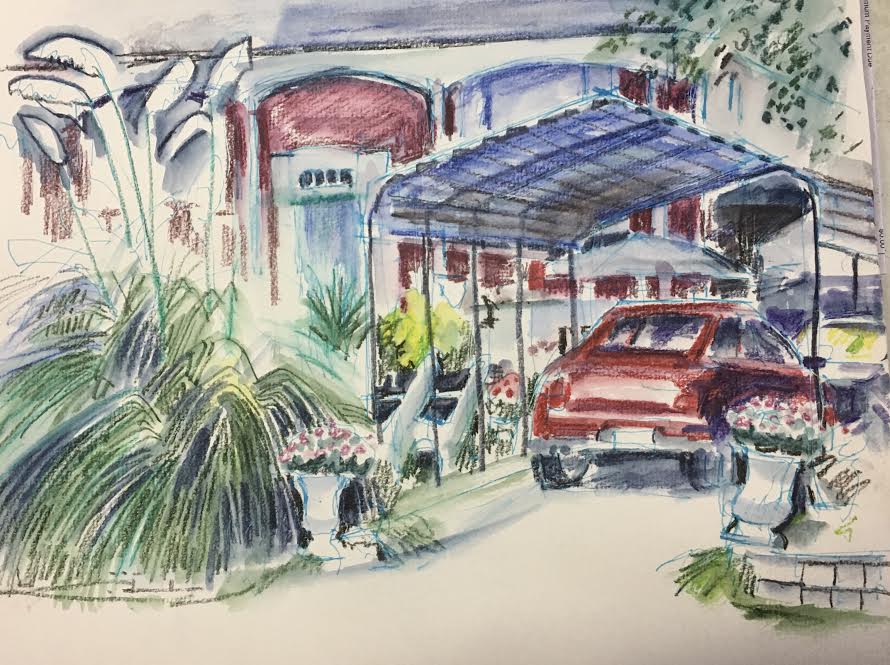The image is a richly detailed and artfully designed colored pencil or charcoal sketch, capturing an inviting scene of a vibrant residential dwelling. The house, possibly a large two-story home or converted apartments, features a white facade with maroon and red accents that bleed together in a fabulously artistic style. The building has curved archways and pillars supporting a distinctive blue corrugated carport, sheltering two cars. One car, prominently displayed in the foreground, is red, while another, partially obscured in the background, appears to be grey.

A lush array of blooming plants and colorful flowers surround the home, adding to its picturesque charm. To the right, red and white flowers sit in elegant grey planters atop a small brick wall. Tall, thin-leaved plants with large, white sheaths of grass, reminiscent of bog cotton, stand to the left. White and yellow flowers intersperse the scene, enhancing the vivid and lively atmosphere. The carport itself is supported by metal poles, beneath which the red car aligns with a detailed depiction showing its rear hatchback.

This captivating artwork, photographed while lying on a surface, combines precision and looseness, illustrating a vibrant blend of nature and architecture in an almost dreamlike, colorful setting.